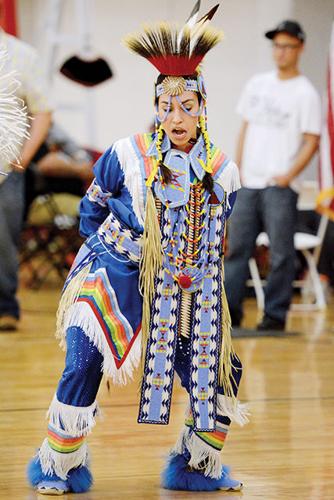The photograph captures a vibrant scene of a traditional Native American dancer, a woman adorned in intricate and colorful attire, performing in a gymnasium with a shiny, light brown hardwood floor. She wears a striking feathered headdress with a red base, splaying out into black-tipped feathers and a gold circular headband with a white band. Her ensemble consists of a blue robe with white fringe along the shoulders and bottom, decorated with a rainbow of colors in diamond shapes and lines. She also dons matching blue pants with two layers of fringe interrupted by rainbow patterns. A long blue ornament dangles from her neck, and she completes her outfit with fluffy blue moccasins. The woman is captured mid-dance, knees bent, arms gracefully positioned behind her back. In the background, two men in white t-shirts and blue jeans, one wearing a black baseball cap and glasses, observe her performance alongside a scattering of folding chairs. The crowd's attire and the setting suggest a community gathering, immersed in the rich cultural display.